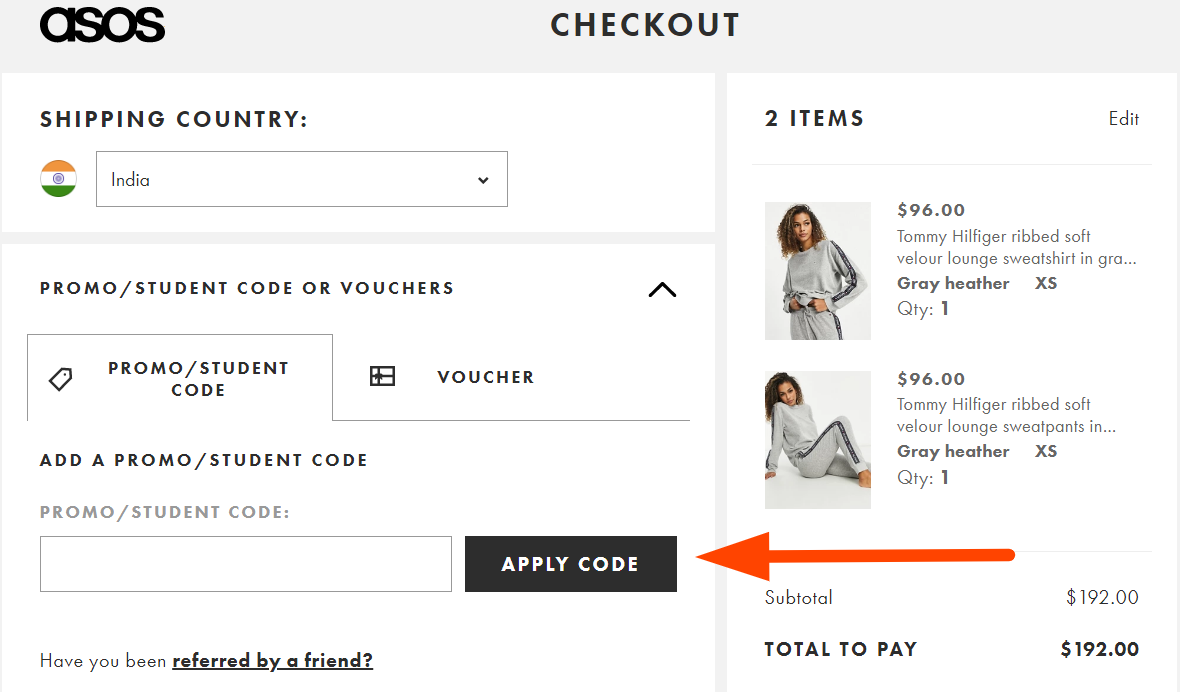At the top of the image, there is a light gray header featuring the ASOS logo in lowercase black bold letters. To the right of the logo, in smaller black capital letters, the word "CHECKOUT" is displayed. Below this header, there is a white rectangular box with the text "SHIPPING COUNTRY" in black capital letters. Directly beneath this, the Indian flag is shown, indicating that the drop-down menu is set to "India."

Further down, there is a section labeled "PROMO / STUDENT CODE or VOUCHERS." This section is divided into two tabs: the first tab is labeled "PROMO / STUDENT CODE," and the second tab, which can be clicked, is for entering a voucher code. Below these tabs, the text "ADD A PROMO / STUDENT CODE" is seen, followed again by "PROMO / STUDENT CODE" with an accompanying text box for code entry. To the right of this text box is a black rectangular button with "APPLY CODE" written in white capital letters. An orange arrow next to this button points towards it, indicating where to click to apply the code.

Further down the page, the text "HAVE YOU BEEN REFERRED BY A FRIEND?" is visible. On the right side of this section, the details of the shopping cart are displayed: the number of items, "TWO ITEMS," the subtotal amount "$192," and the "TOTAL TO PAY" of $192.